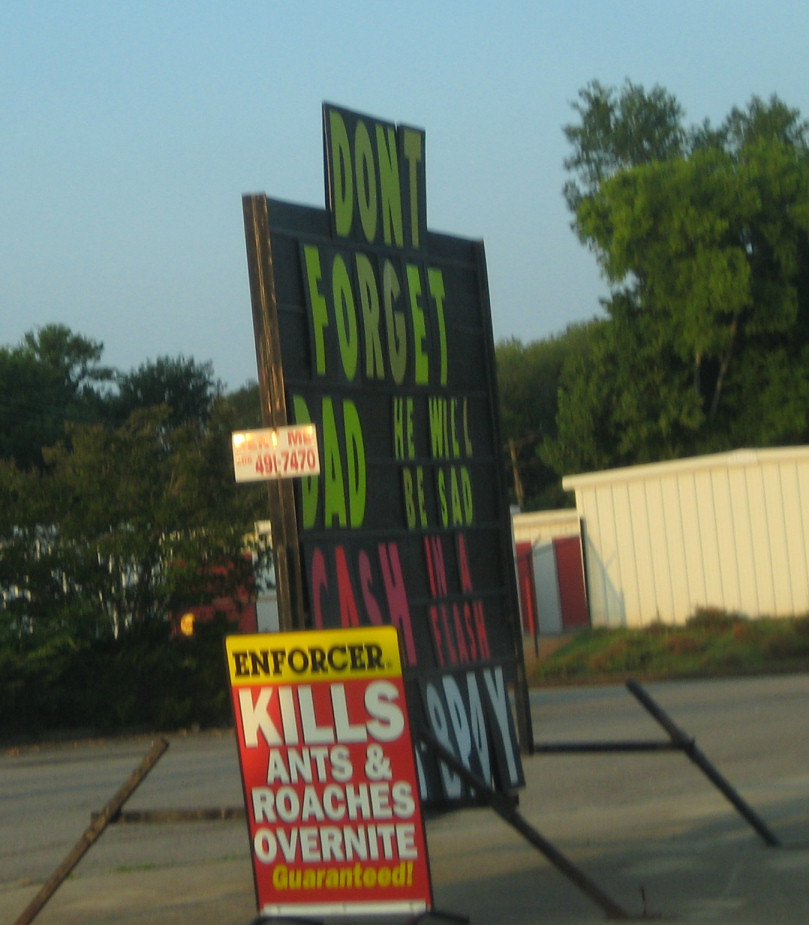An image showcasing an intriguing outdoor advertisement setup. The scene, seemingly captured in the afternoon with natural sunlight casting a mild shadow, features a pair of signs positioned on the ground near a retail area. The backdrop includes a cream-colored building and other structures partially obscured by distant trees.

The prominent sign, styled like a billboard though situated at ground level, has a black background with bold, green, capitalized text that reads: "DON'T FORGET DAD, HE WILL BE SAD." Below this, in striking red letters, the message "CASH IN A FLASH" is displayed, hinting at a quick monetary service, possibly a payday loan. The sign also includes a business phone number.

Adjacent to this large sign is a smaller, vibrant advertisement in red, yellow, and white, depicting an offer: "Enforcer kills ants and roaches overnight guaranteed," emphasizing a pest control solution.

The combination of these signs suggests a multifaceted advertising approach, probably aimed at capturing the attention of shoppers—potentially promoting Father's Day gifts alongside fast-cash financial services and pest control products.